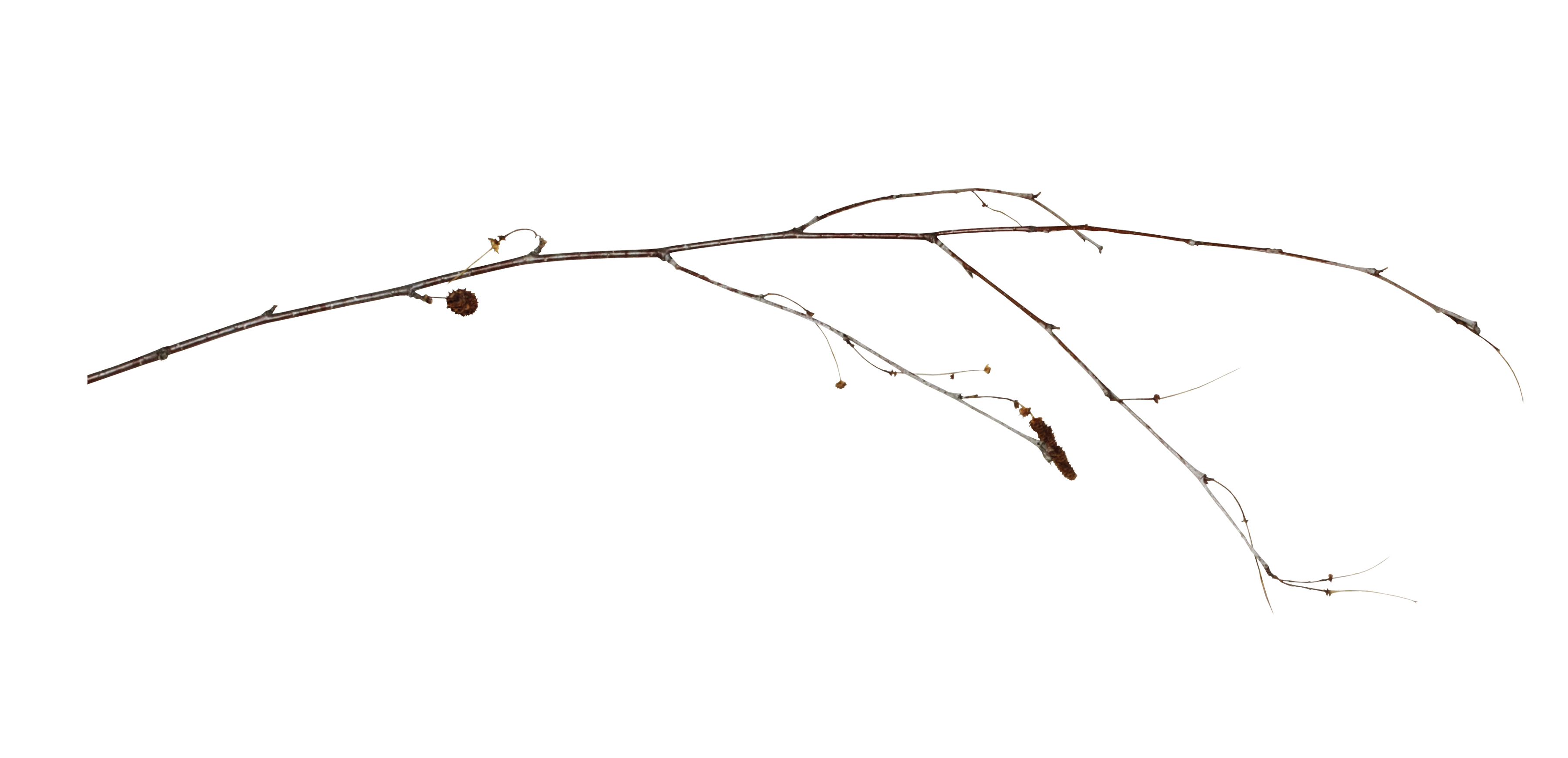The image depicts a thin, horizontally positioned branch set against a completely white background. Extending to the right, the branch starts with a series of protruding shoots: one at the bottom bearing a small brown acorn or nut. Above this, a thinner shoot emerges to the right, followed by another on the left, and then another to the right. One of these minor shoots has a leaf-like projection, while another has a curling twig forming a sideways teardrop shape. Near the end of the main branch, a longer shoot extends downward to the bottom right, displaying several small black seeds clustered together. The overall structure is characterized by its delicate, wispy twigs and various buds, adding intricate details to the otherwise singular main branch.